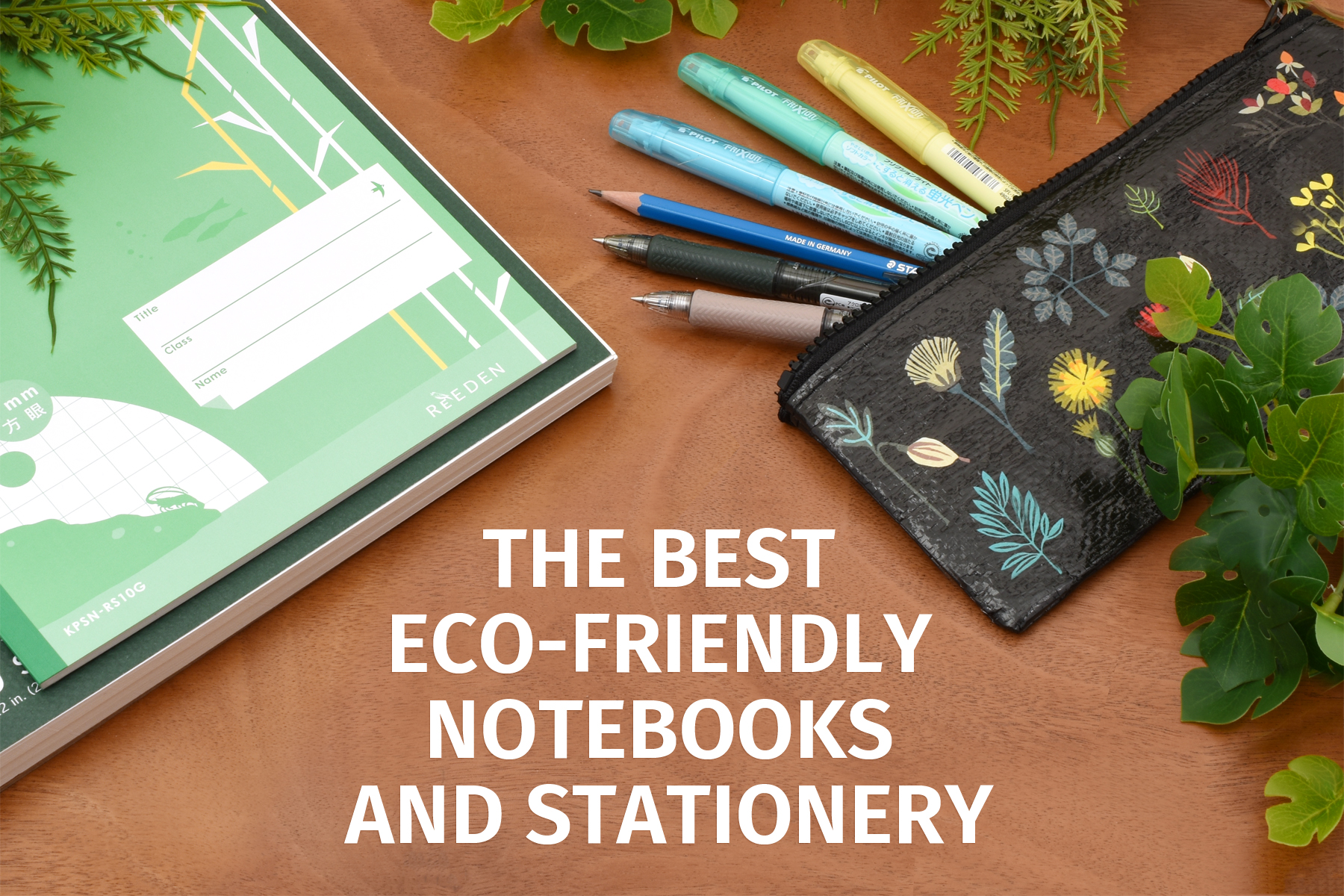The image portrays an advertisement featuring an assortment of eco-friendly notebooks and stationery, displayed on an orange wood table. On the left side, there are two notebooks: the top one is green with white and yellow bamboo designs and a space for a name in the bottom right area, along with a white globe on the left side. Beneath it lies a dark green cover notebook. To the right, there is a black pencil pouch adorned with floral patterns in blue, yellow, red, and white. The pouch contains six writing utensils arranged left to right: a yellow marker, two blue markers, a blue pencil, a black gel pen, and a light purple gel pen. Surrounding the items, green leaves and plants are scattered, appearing at the top left corner, the middle, and the top right corner. The middle bottom of the image features bold white text that reads “The best eco-friendly notebooks and stationery.”